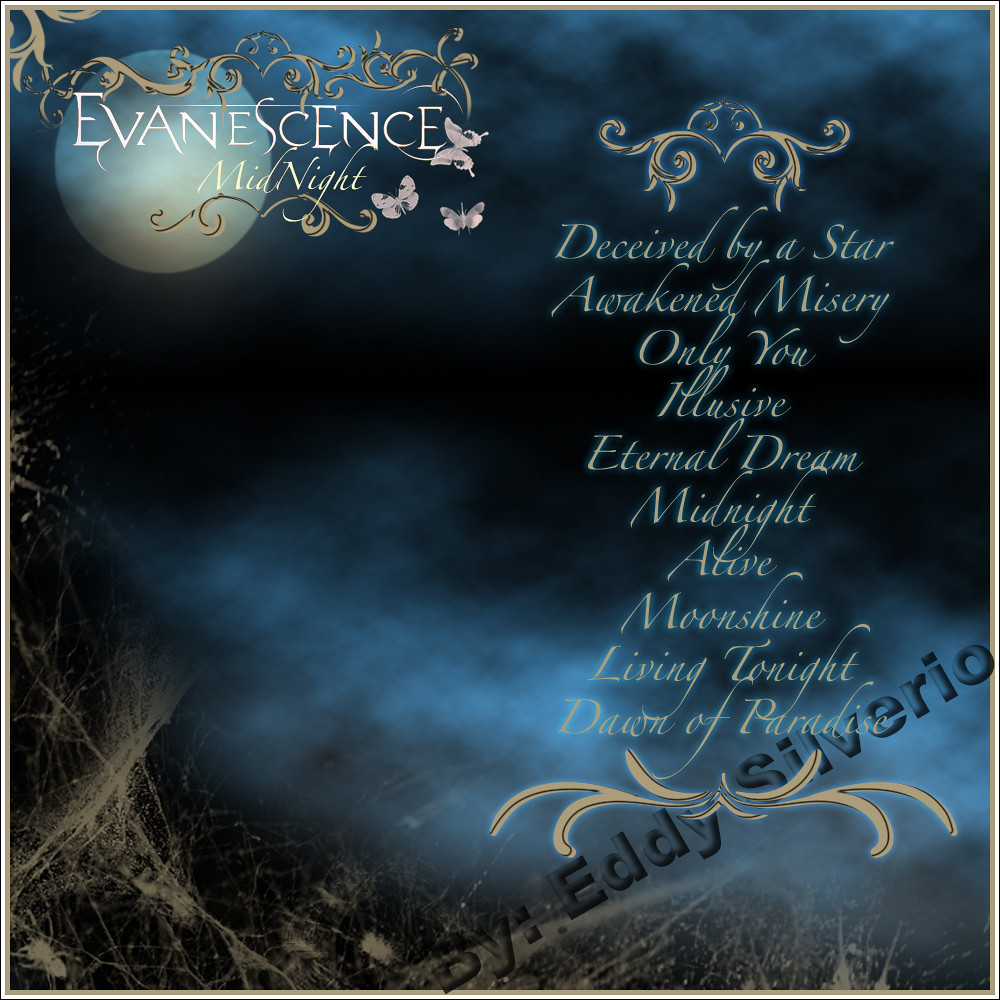The image appears to be a cover for an album, possibly a magazine or book, or an advertisement poster, with a dark navy blue and almost black background, suggesting a night sky. In the upper left corner, there are some beige-colored etchings alongside the text "Evanescence, Midnight" in white letters. The scene is adorned with butterfly symbols and the moon, contributing to the nocturnal theme. Light blue clouds are visible, adding depth to the sky. Below the title, there's a list resembling a tracklisting, which includes: "Deceived by a Star," "Awakened Misery," "Only You," "Illusive," "Eternal Dream," "Midnight," "Alive," "Moonshine," "Living Tonight," and "Dawn of Paradise." The lower right corner of the cover features the name "By Eddie Silverio." The background also includes faded images of dried plants or sticks, enhancing the eerie, dreamlike atmosphere.